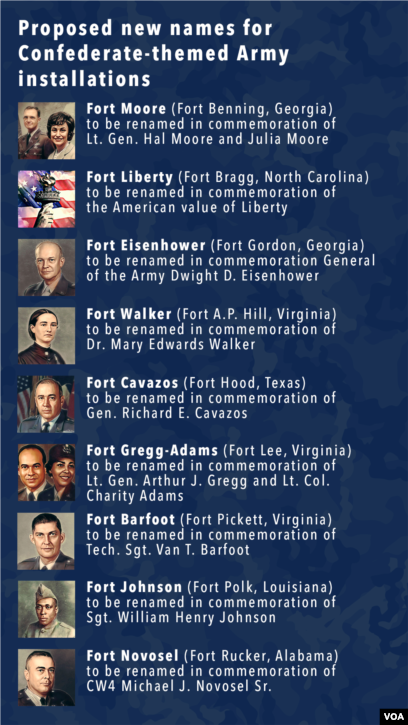The image is an infographic poster titled "Proposed New Names for Confederate-Themed Army Installations," with a navy blue background and a tall rectangular layout. At the top, in white text, it lists proposed new names for nine forts, each accompanied by a photo or painting. The entries provide detailed information about each fort's namesake:

1. **Fort Moore** (Fort Benning, Georgia) - To be renamed in honor of Lieutenant General Hal Moore and Julia Moore, with their portrait beside it.
2. **Fort Liberty** (Fort Bragg, North Carolina) - To be renamed to symbolize the concept of liberty, depicted by a hand holding a torch in front of an American flag.
3. **Fort Eisenhower** (Fort Gordon, Georgia) - To be renamed for General Dwight D. Eisenhower.
4. **Fort Walker** (Fort AP Hill, Virginia) - To be renamed for Dr. Mary Edwards Walker.
5. **Fort Cavazos** (Fort Hood, Texas) - To be renamed in commemoration of General Richard E. Cavazos.
6. **Fort Greg-Adams** (Fort Lee, Virginia) - To be renamed for two individuals at different ranks, possibly a general, and a lieutenant colonel.
7. **Fort Barfoot** (Fort Pickett, Virginia).
8. **Fort Johnson** (Fort Polk, Louisiana).
9. **Fort Novosel** (Fort Rucker, Alabama).

In the lower-right corner, a black box with white text says "VGA." The poster offers a visual guide aimed at informing about the renaming initiative, detailing each proposed name and its significance.